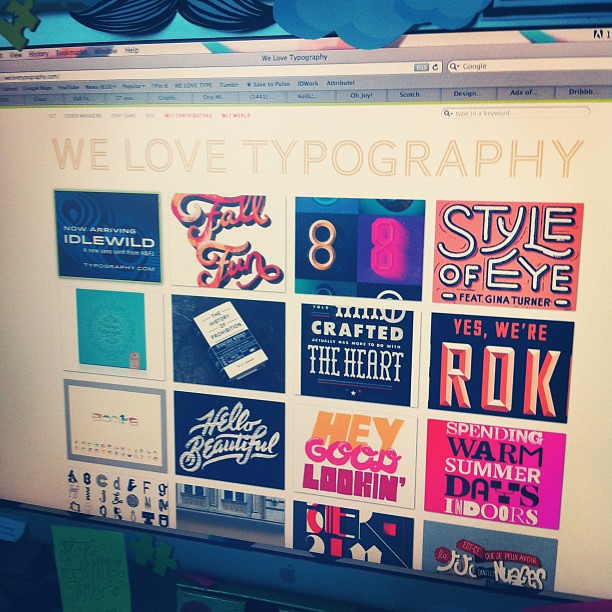In this full-color photograph, which appears to be a computer screen with multiple tabs at the top, there is a prominent sign reading, "We love typography, like photography only it's typography." The background is a light beige, slightly darker than the beige lettering of the sign. Below this sign are several rows and columns of colorful tiles, each displaying different phrases in various typography styles. 

The top left tile is blue with white text saying, "Now arriving Idlewild." To its right is a tile with cursive red and yellow text that reads, "Fall Fun." Next to that, there is a tile featuring the number "88," where one "8" is in gold and the other in neon pink. Following this is an orange tile with white text that says, "Style of Eye feat. Gina Turner."

The subsequent rows contain more diverse and colorful tiles. Phrases visible here include "Crafted the Heart," "Yes, we’re rock okay," "Hello Beautiful," "Hey, Good Looking," and "Spending warm summer days indoors." Each tile features unique and striking typography, making the entire display a vibrant collage of fonts and colors celebrating the art of typesetting.